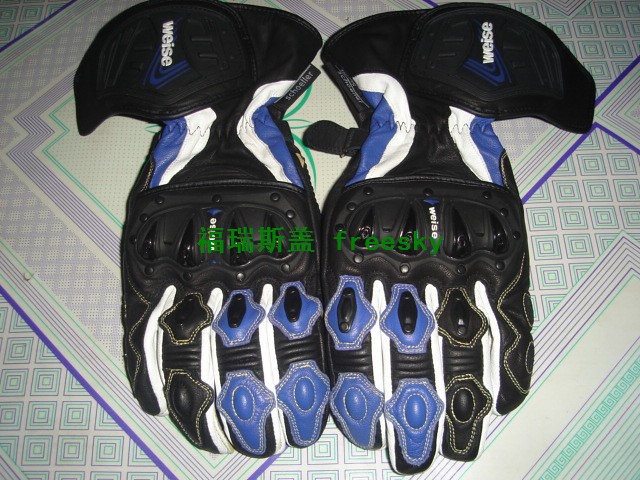This professional promotional photo showcases a pair of motorsport gloves, which could also be used for activities such as motorcycling or snowboarding. The gloves prominently feature a combination of black, white, and cobalt blue colors. Each glove has distinct detailing: the left glove has writing in an Asian language, while the right glove bears the word "freeski" or "freesky" without any spacing. The gloves are made of leather, with extra padding and intricate patterns on the knuckle areas for added protection. Notably, the brand name "Weise" (spelled W-E-I-S-E) is printed on the wrist area with zigzag stitching. The background of the photo features a vibrant, 80s-inspired graphic pattern combining lavender, kelly green, and ivory in a mix of stripes, diamonds, polka dots, and checkered designs, adding an eye-catching contrast to the gloves.